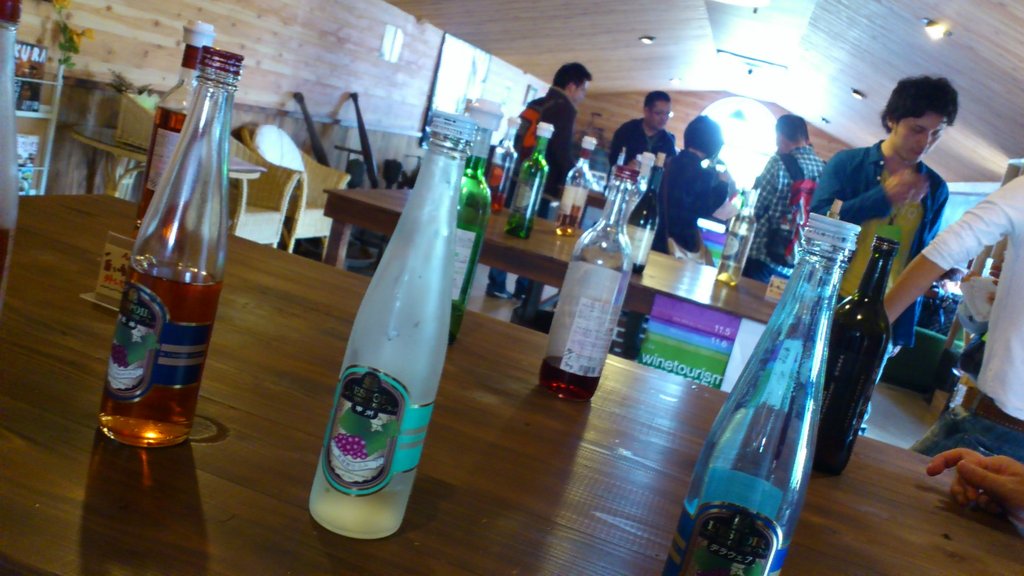The image depicts a rustic, indoor setting reminiscent of a winery or upscale tasting room, characterized by its extensive use of wood in the walls, floor, and vaulted ceiling. In the foreground, various large bottles with minimal liquid content are neatly arrayed on a wooden table, suggesting a wine or alcohol tasting event. Throughout the room, people are engaged in animated conversations, with some examining specific bottles and others holding cups of tasting samples. In the background, additional tables share a similar setup, with a sign on one of them indicating "wine tourism." The space is brightened by natural light streaming through a large window at the back, further enhancing the warm, inviting ambiance of the wood-accented environment. Shelves on the left-hand side display extra bottles, and chairs are arranged along the walls for seating.